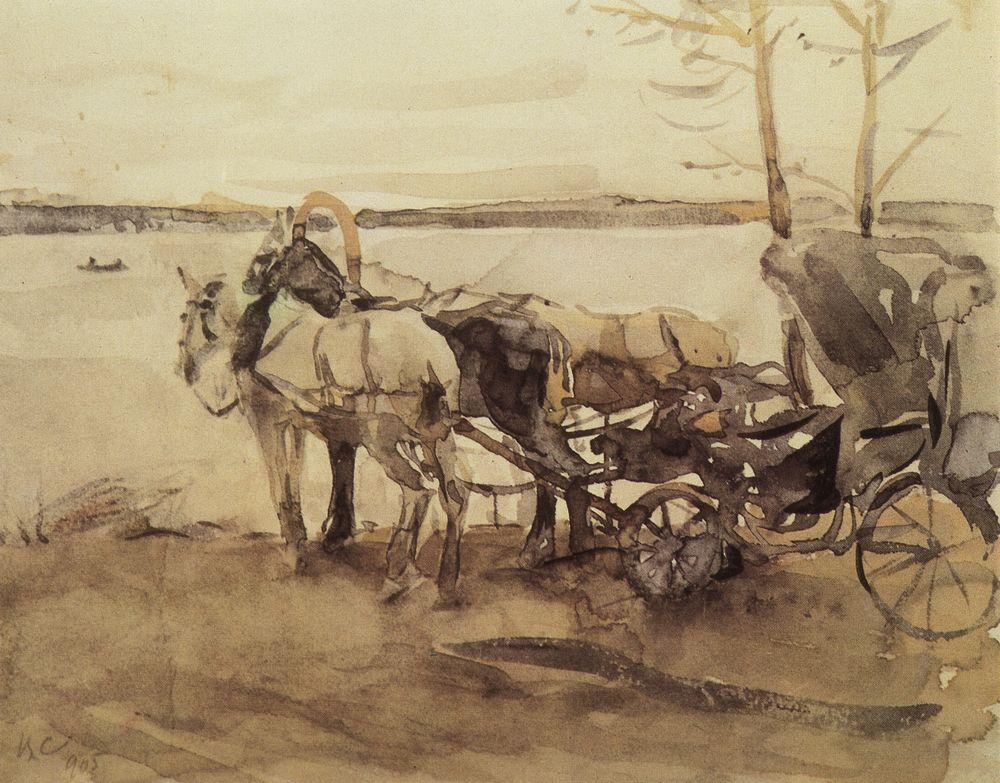This sepia-toned watercolor painting depicts a tranquil scene of a horse-drawn carriage by the riverside. The painting uses a palette of brown and gray tones, giving it a nostalgic, antiquated feel. In the foreground, there is an old 19th-century-style carriage being pulled by three horses, their wooden wheels and harnesses detailed yet subtle in the sepia wash. These horses, appearing contemplative, face a wide, light-colored body of water, possibly a lake or river, reflecting the soft glow of what seems to be a setting sun. Alongside the carriage are two small trees, adding to the sparse yet serene landscape. The terrain around them is barren and flat, creating a sense of open space and stillness. In the distant background, across the body of water, lies a mass of flat land, emphasized by an orange-brown gradient that hints at an approaching dusk. A small canoe can be seen far off on the water, adding a final touch of quiet melancholy to the scene.